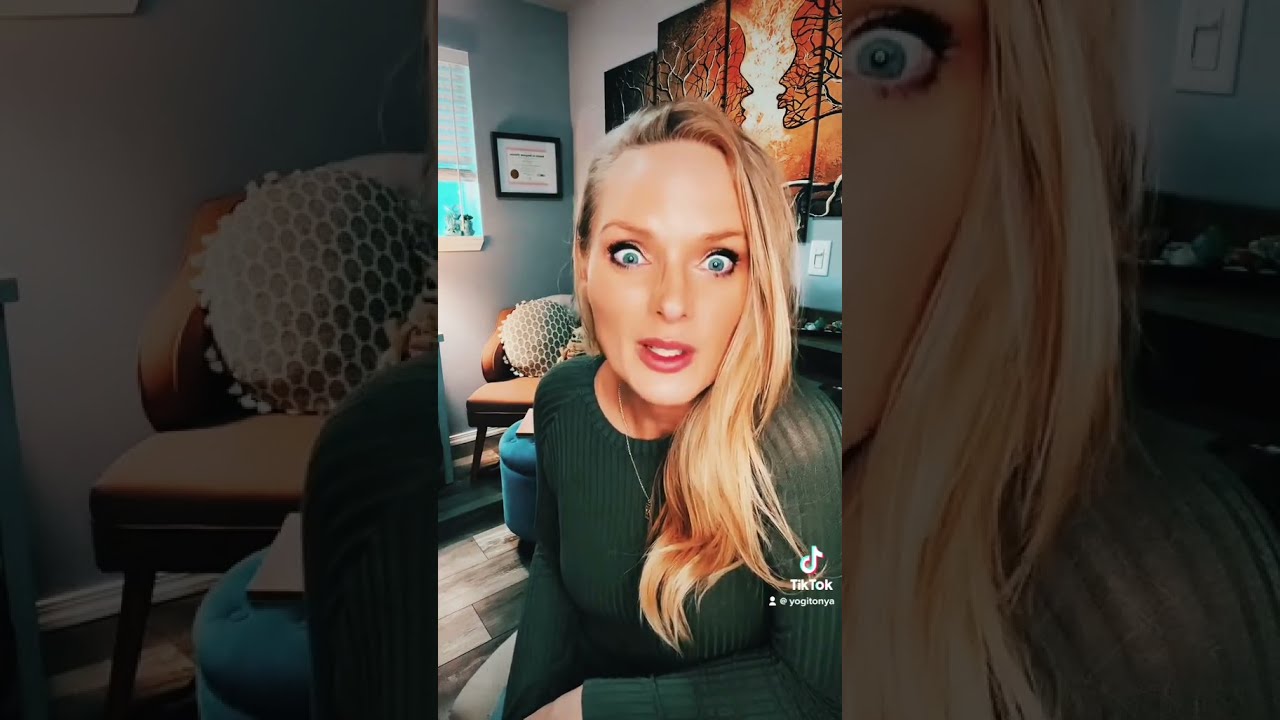The image is a detailed screenshot of a TikTok influencer, a Caucasian woman likely in her 30s, with blonde highlighted hair and striking bright blue eyes, which are wide open in a surprised expression. She is seated, possibly in her home office, amidst a setting that includes an abstract painting in orange and white depicting two people kissing and a degree in the back corner. She wears a long-sleeved green sweater with ribbed texture, adorned with the TikTok logo near her shoulder. Her lips are painted in a vivid red lipstick, complemented by heavy black mascara. The background of the image is split, with the left third showing an enlarged portion of her background furniture and the right third featuring a blown-up section of her face, highlighting her wide eye and hair. The image's composition centralizes the woman's comically shocked expression, adding a dynamic and engaging visual element.